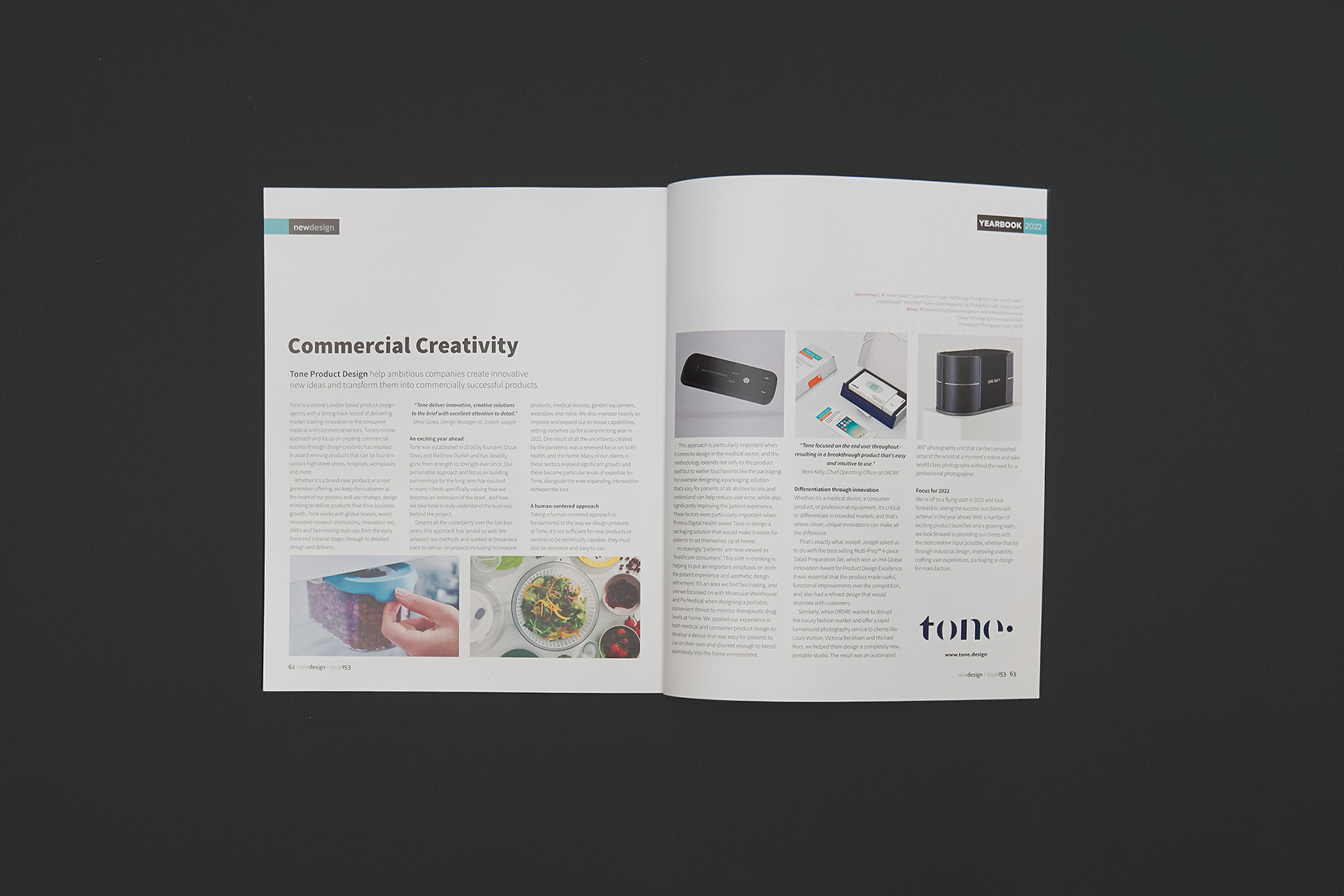The photograph features an open magazine centered on a large, dark gray background that might be a tabletop or a digitally-added backdrop. The magazine's left page prominently displays the heading "commercial creativity" in bold letters, followed by several paragraphs of text discussing how ambitious companies can generate innovative ideas and transform them into commercially successful products. This page also includes two inset color photographs near the bottom: one showing a hand placing a container of berries with a blue top into a refrigerator, and another depicting bowls with various food items, possibly a salad and side dishes. The right page of the magazine is titled "Yearbook 2022" in the top right corner and contains three photographic illustrations. The first image shows a black rectangular tool with silver screws or buttons, the next is of two white boxes with different colored labels, and the third appears to be a black cylindrical case, possibly a jewelry box. There are descriptive paragraphs beneath each image, although the text is difficult to read at this size. The bottom right corner of the right page features the word "tone" written in lowercase letters.